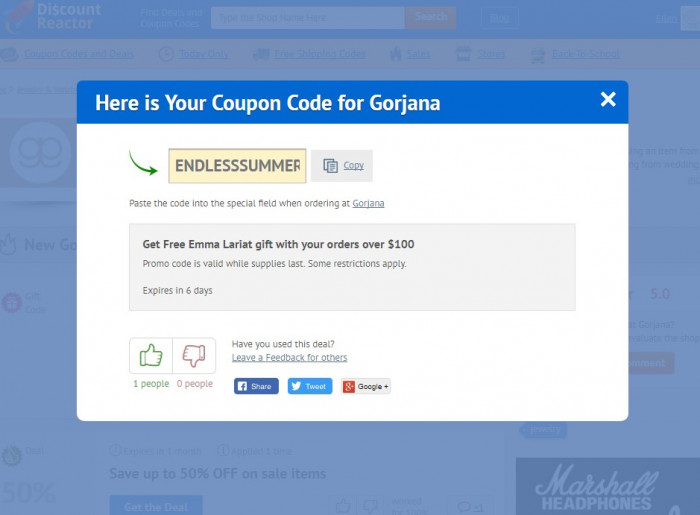This image depicts a promotional webpage designed to attract customers with various offers and discounts. At the top left corner, a search bar provides an easy way to navigate the page. There are several categories displayed, including "Coupons," "Codes and Deals," "Trade Today Only," and "Free Shipping."

A centrally-located section showcases a coupon for Gojourner under the banner "Back to School," accompanied by the phrase "Endless Summer." It instructs users to copy and paste the provided promo code into a special field when placing an order at Gojourner. The promotion offers free gifts and malaria prevention kits for orders exceeding $100, with the code valid while supplies last and expiring in six days. It notes that some restrictions may apply.

Below the promotional content, the page encourages users to leave feedback on their orders and share their experiences via Facebook, Twitter, or Google. This visually engaging and informative layout aims to enhance users' shopping experience and drive engagement.